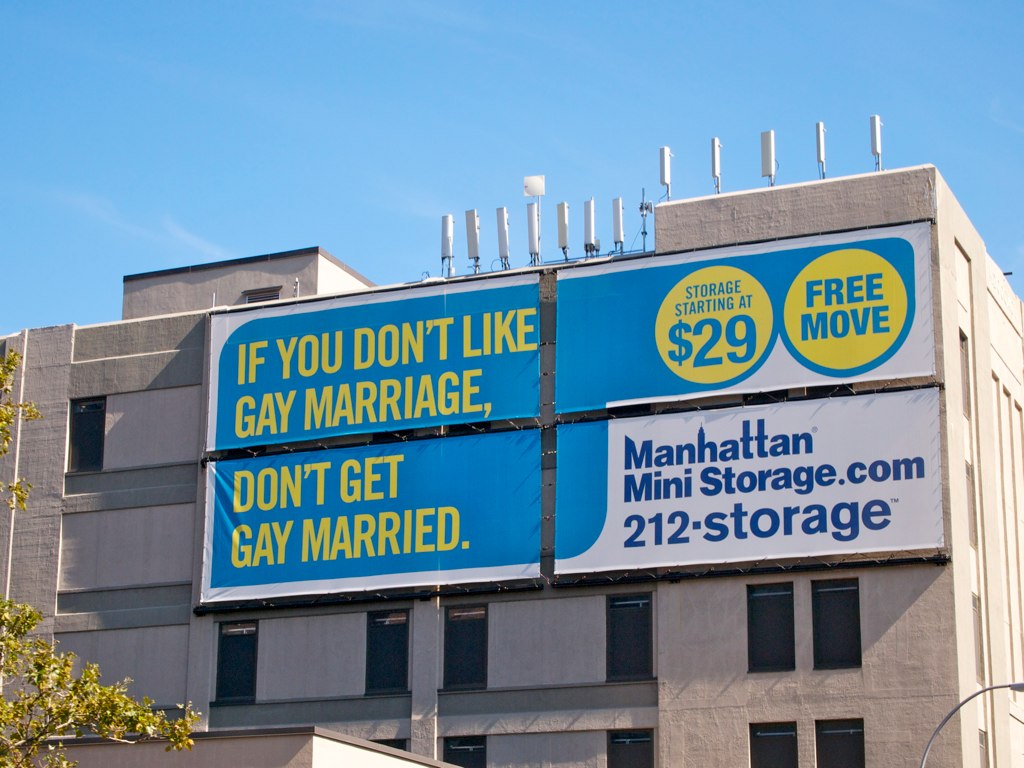In the image, a light blue sky dominates the background, adorned with lines of white clouds predominantly clustered toward the top left corner. Central to the scene is a white building, its façade striking against the serene sky. The structure features multiple windows, all obscured by black curtains, giving it an enigmatic appearance. Adorning the top section of the building are four posters. The two upper posters collectively carry a thought-provoking message: "If you don't like gay marriage," followed by, "Don't get married," both prominently written in yellow text against a blue background. Additionally, the top-right poster advertises storage services with the text, "Storage starting at $29." This juxtaposition of messages lends a unique, layered character to the outdoor scenery.